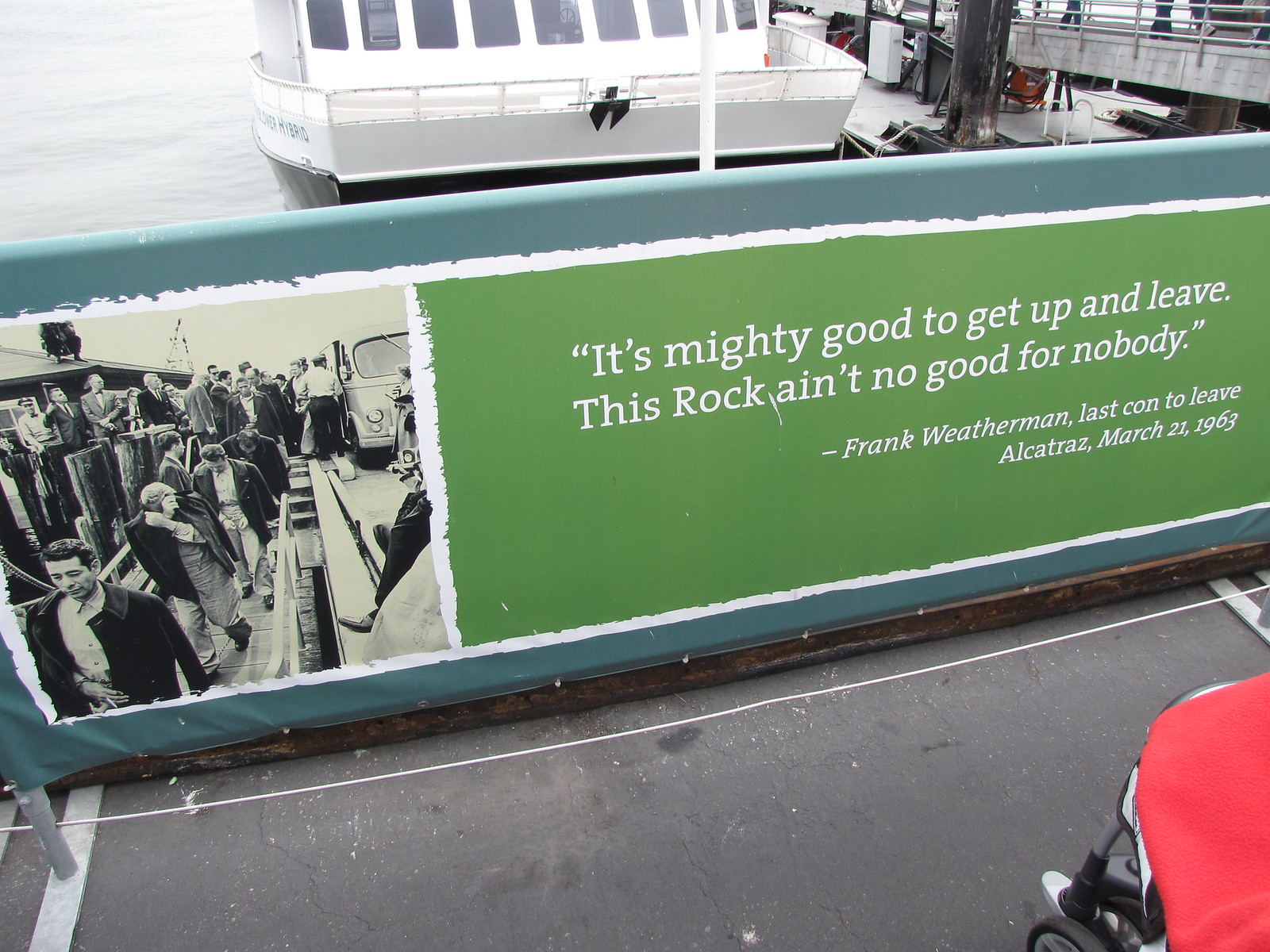The photograph captures a detailed scene outdoors during the daytime, focusing on a long, green and white banner sign displayed horizontally across a guardrail by a pier or dock. The banner prominently features a historic black-and-white photograph on its left side, depicting a group of prisoners walking down a gangway or plank. The text on the sign, in white against the green background, quotes Frank Weatherman, the last convict to leave Alcatraz: "It's mighty good to get up and leave. This rock ain't no good for nobody. Frank Weatherman, last con to leave Alcatraz, March 21st, 1963." In the background, a white boat with a black hull, resembling a ferry, is docked by the water, while people can be seen walking along the dock. The foreground includes a gray floor and a partial view of a red covering or cloth. To the top right, another gangway is visible, and a person dressed in red stands near the banner, possibly reading it. This image captures the essence of a historical Alcatraz tour setting, evoking a strong sense of the island’s past as a prison.